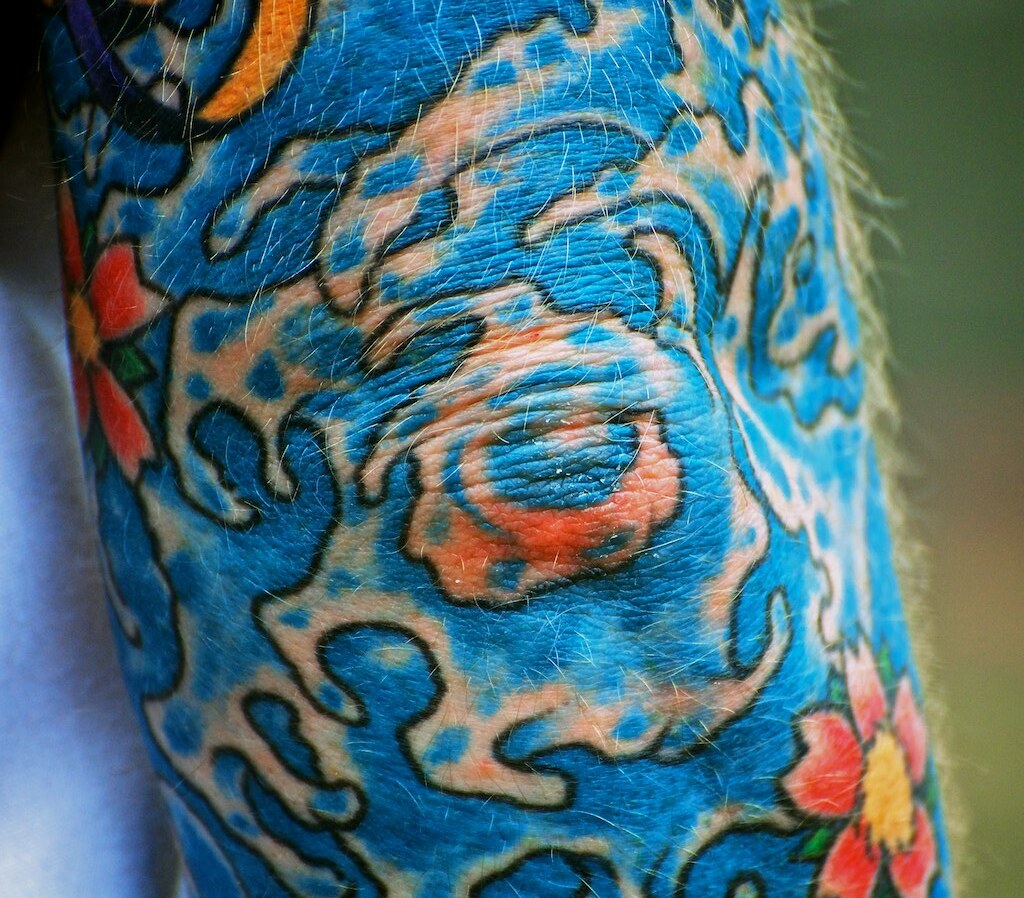The photograph captures a close-up view of a tattooed arm, likely the elbow based on the protruding joint and some wrinkles. The arm, heavily adorned with intricate blue waves and outlined in black, stretches diagonally from the top left to the bottom right of the image. The tattoo prominently features a striking design of waves that curve and swirl around the arm, particularly emphasizing the joint area. Two vibrant pink flowers with orange centers embellish the design, positioned at the upper left and lower right corners of the tattoo. Additionally, there's a red flower with a yellow center visible at the bottom right corner of the image. The tattoo is detailed with blue shading inside an orange splotch at the joint. Around this complex art are numerous gray hair follicles, adding texture to the skin. The background of the photograph is blurry, displaying a mix of green, brown, and yellow hues, indicating a shallow depth of field that keeps the intricate tattoo in sharp focus.